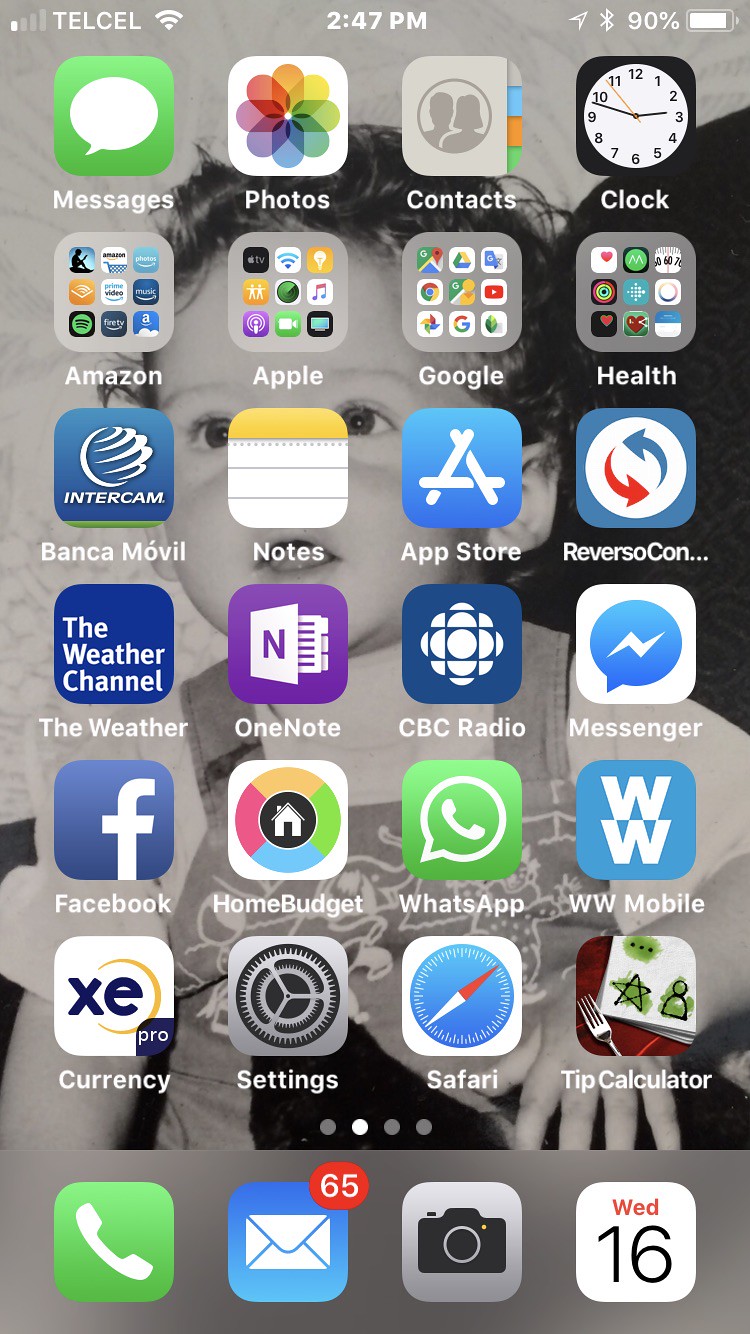A screen capture of an Apple iPhone home screen, showcasing a variety of icons and apps neatly arranged. The top left corner indicates the cellular provider as Telcel with a current time of 2:47 PM and a battery level at 90%. The home screen features several standard app icons such as Messages (showing 65 unread texts), Photos, Contacts, and Clock. 

Additionally, there is a folder containing multiple apps which include Amazon, Apple, Google, and Health. Other notable app icons visible are for a banking app, Notes, the App Store, The Weather Channel, OneNote by Microsoft, CBC Radio, Facebook Messenger, and Facebook. The screen capture also reveals that the default browser is Safari.